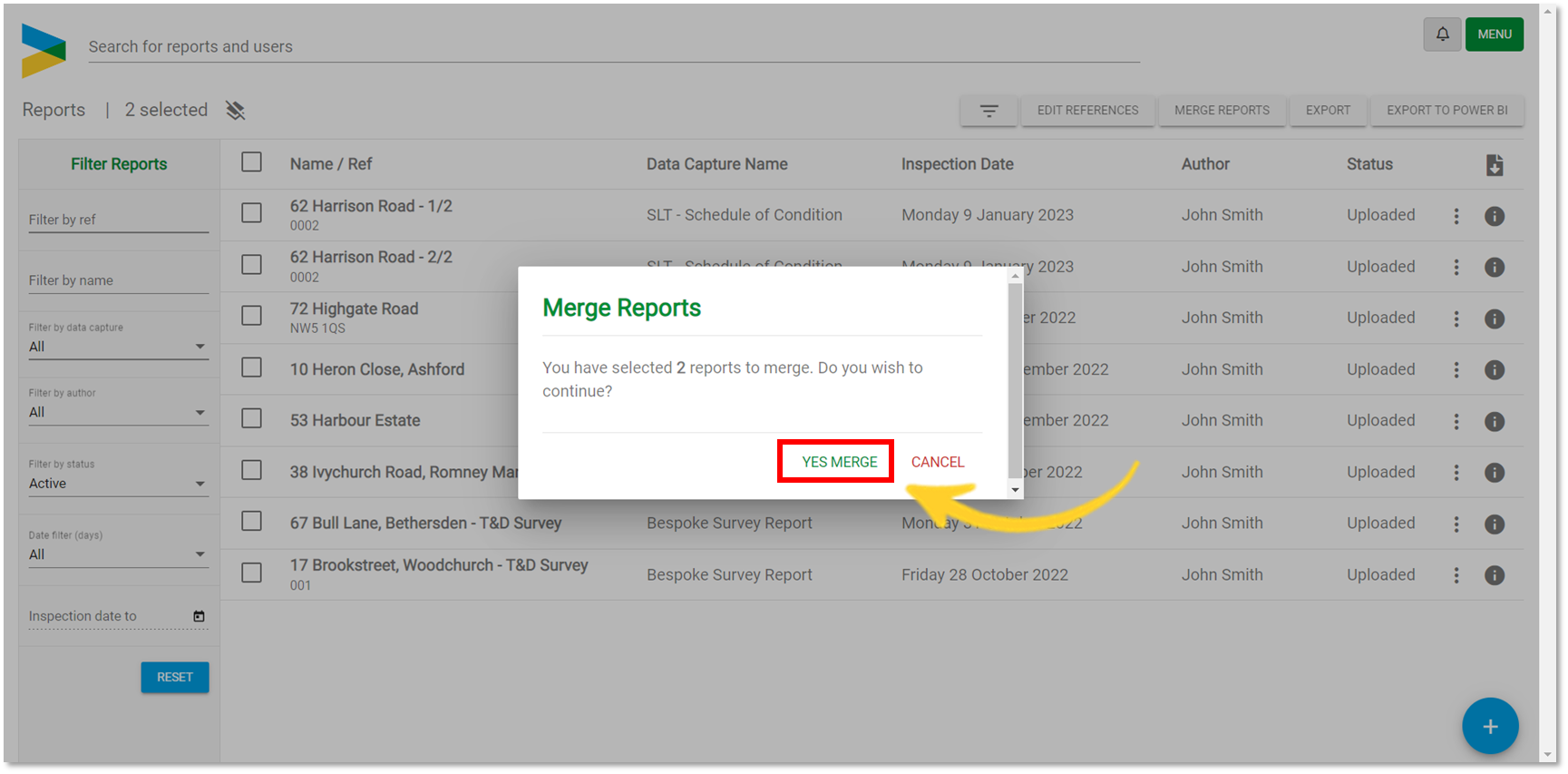The image depicts a digital report interface. In the top left corner, there is a search bar labeled "Search for reports and users." Adjacent to this, a distinctive, sideways "V" logo with blue and yellow colors marks the left side of the header. Below, a section titled "Filter Reports" features various filtering options.

In the center of the page, a prominent white box stands out with the header "Merge Reports." It contains the message, "You have selected two reports to merge. Do you wish to continue?" A red-outlined button labeled "Yes, Merge" is highlighted with a yellow arrow pointing to it, indicating the primary action. Beside it to the right, there is an option to "Cancel."

In the top right corner, a green notification bell and a menu icon are visible, likely for additional settings or alerts. Toward the bottom of the interface, a blue button labeled "Reset" allows users to reset the filters or selections.

The main body of the interface consists of numerous lines representing different entries, each with empty checkboxes that users can select. Columns are labeled to display information such as "Author" and "Status." In the bottom right corner, a small circle with a cross in the center serves as a closing or exit button for the section.